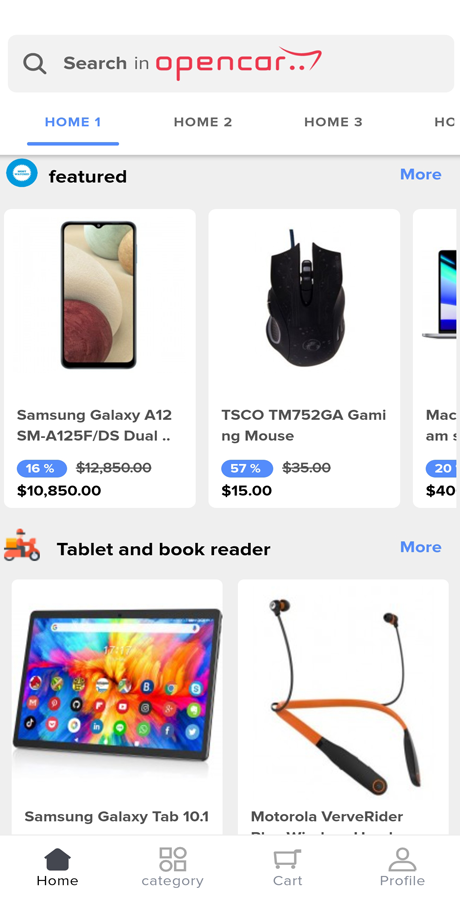This image showcases a close-up view of an open car website. At the top, a light gray search bar extends horizontally across the screen, inviting users to "search in open car." However, both the left and right sides of the website are partially cropped out of the image. Directly below the search bar, there are three items displayed side by side in the featured section. Starting from the left, the first item is a Samsung Galaxy A12 (Model SMA125F/DS), priced at $10,850. Next to it, on the right, is a computer mouse priced at $15. The final item in this row appears to be a laptop, but it is partially cut out of the image, making its details unclear. Further down the page, there is the "tablet and book reader" section. Within this section, we see a tablet on the left, and to its right, a pair of headphones.